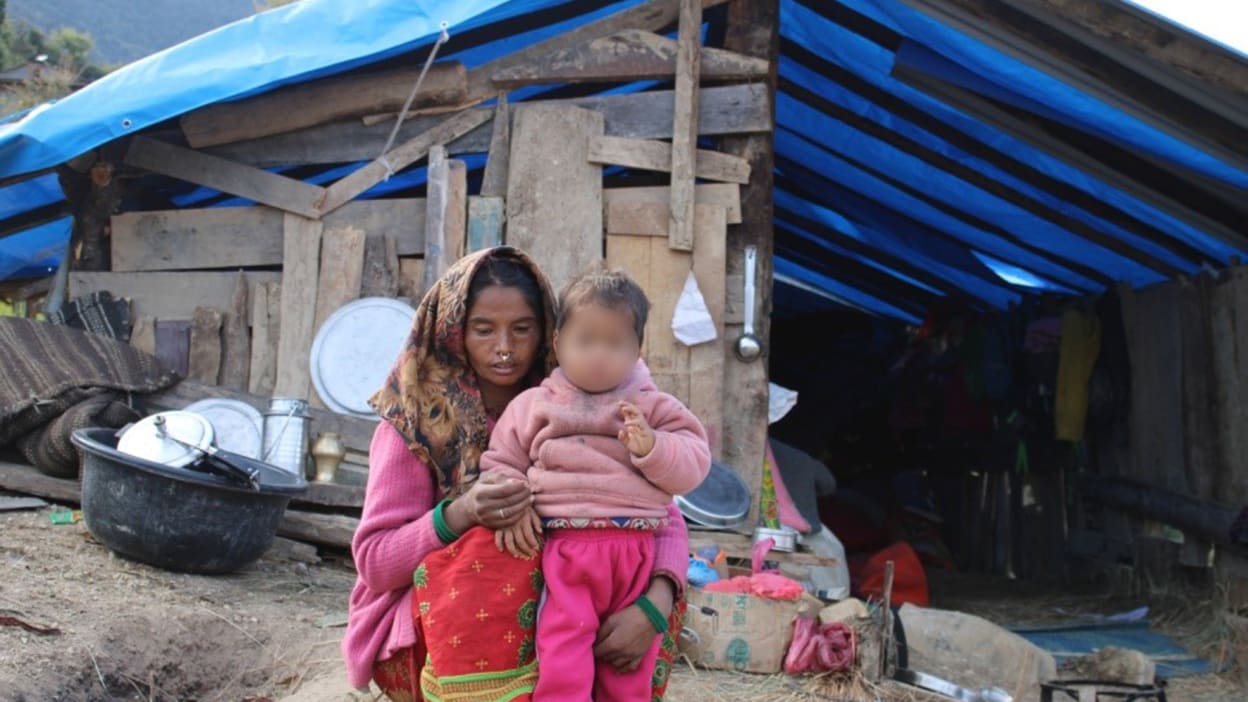In the foreground of the image, a woman is seen squatting, holding a young child in front of her. The woman uses her right hand to grip the child's right arm while her left hand wraps around the child's leg, gently pulling her back. The child, who wears a dull pink sweater and bright neon pink pants, has her face blurred out. The woman, with darker brown skin and black hair, has a nose ring that connects both nostrils and a brown head wrap adorned with black flowers. She is dressed in a long-sleeve pink sweater with green sleeve ends and a red apron-like dress with green patterns.

The backdrop presents a makeshift, ramshackle dwelling composed of haphazardly fastened wooden planks. A blue tarp serves as a rudimentary peaked roof, giving the structure a tent-like appearance. The left half of the shack is partially covered, while the right side is completely open, exposing the interior and reinforcing the rough, improvised nature of their shelter. Various items are scattered around the immediate vicinity.